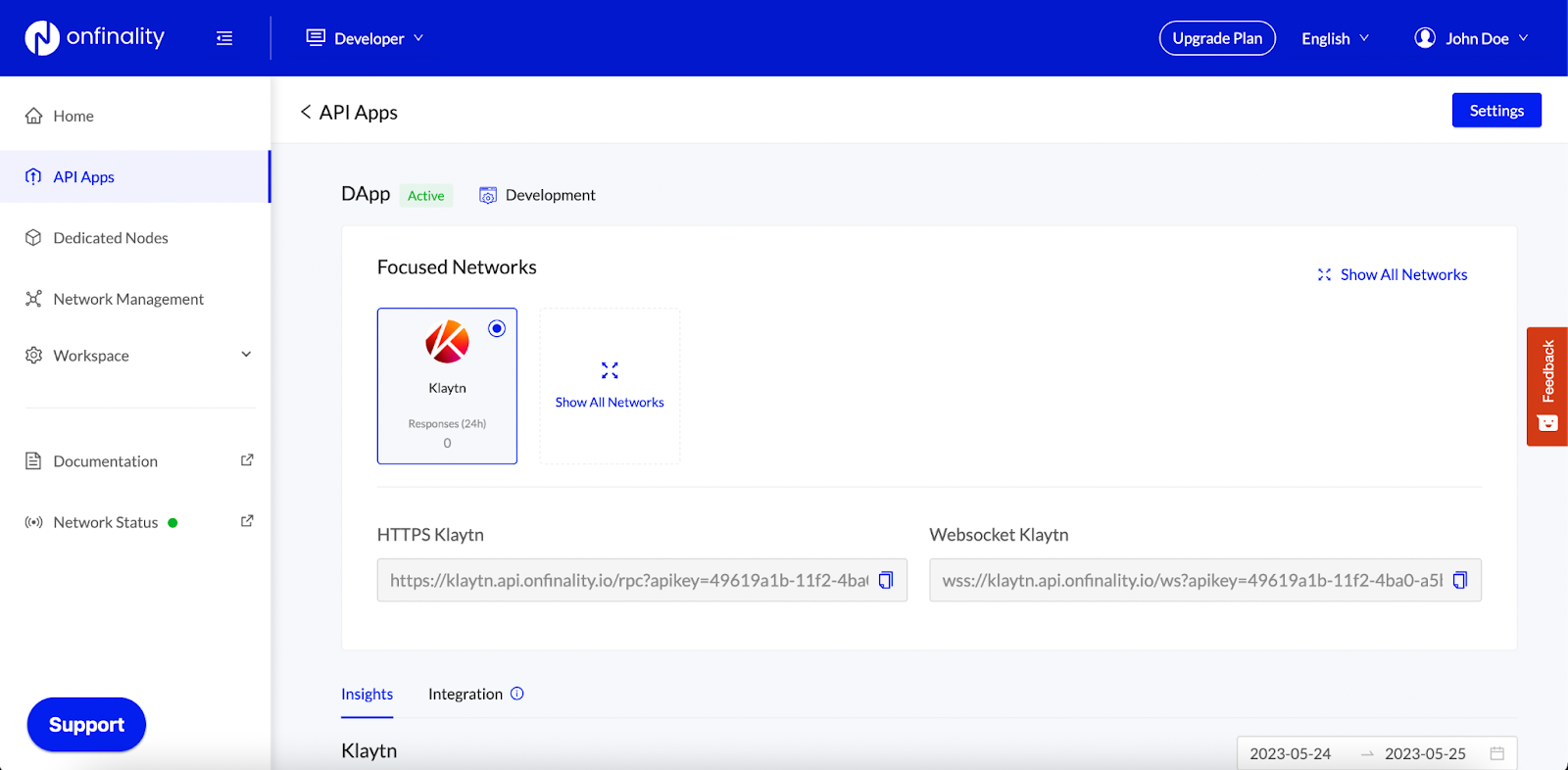The image depicts an interface of a developer's upgrade plan on Finality. The focal point of the display is the "Upgrade Plan" section, featuring an organized layout with several functional areas:

1. **First Circle**: A prominent section titled "John Doe" is displayed, indicating user details or account information.
2. **Left Column**: This menu showcases a variety of functionalities including:
    - Home
    - API Apps
    - Dedicated Nodes
    - Network Management
    - Workspaces
    - Documentation
    - Network Status

3. **Bottom Left**: A panel listing supported items, which include:
    - API App Settings
    - D App (presumably indicating decentralized applications)
    - Active Development
    - Focus Network
    - Show All Networks

4. **Interactive Squares**:
    - One square labeled "Claim" with a response count of 2500.
    - Another square enabling users to "Show All Networks."

5. **Text Details**: The panel includes specific connectivity details with:
    - HTTPS URL: `https://clinton.upi.on.finality.io/RPC?API=49619A1B-11F2-4BA`
    - WebSocket URL: `wss://clinton.upi.on.finality.io/WS?API=49619A1B-11F2-4BA08-85L`

6. **Insights and Integration**: The bottom left corner features a textual remark, "Clinton, that guy is just great," suggesting an acknowledgment or accolade.

7. **Date Stamps**: The bottom right indicates two dates, "2023-05-24" and "2023-05-25," which could relate to updates, modifications, or usage logs.

Overall, the image illustrates a comprehensive and neatly arranged developer interface on Finality, showcasing various tools, user information, connectivity details, and pertinent dates.